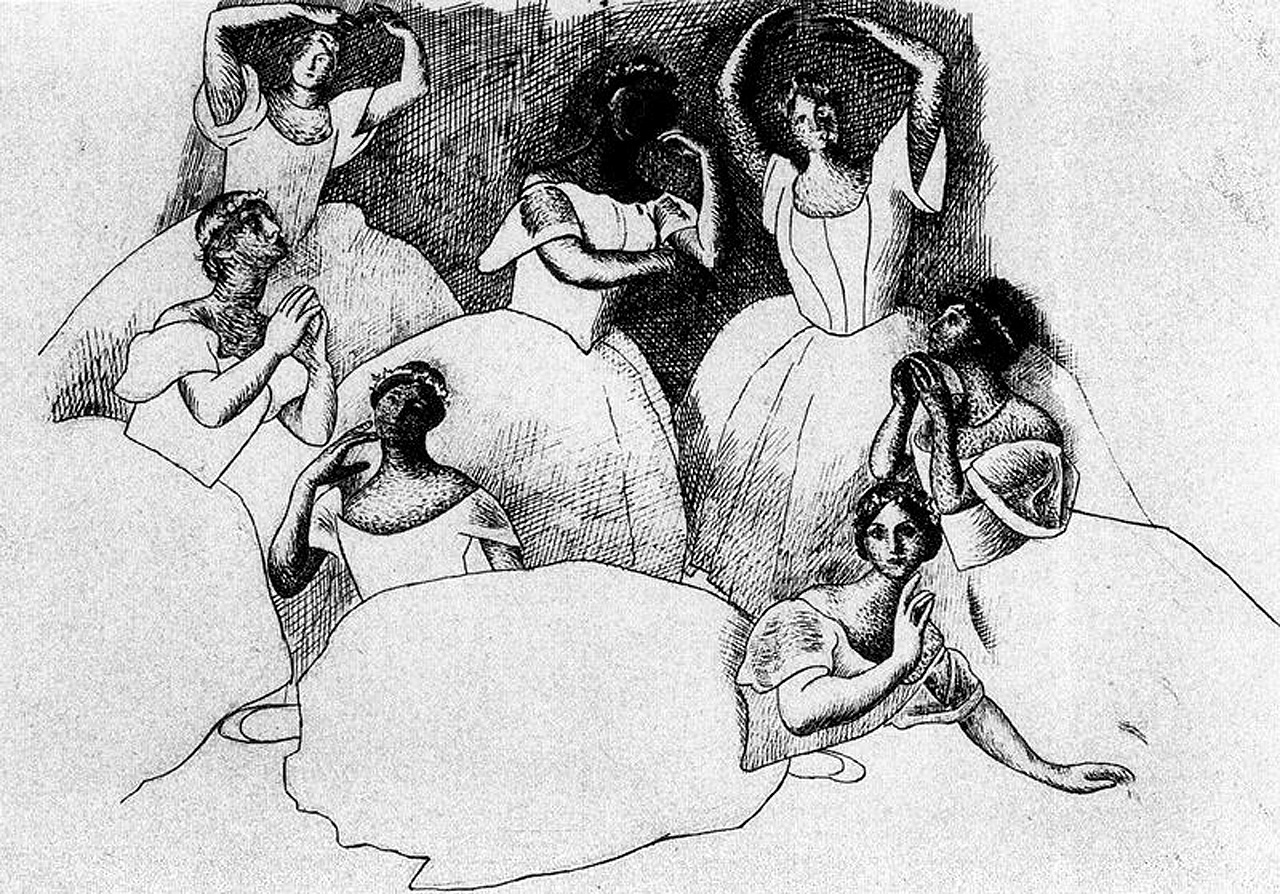The detailed black and white sketch showcases seven elegantly drawn ballerinas, all clad in flowy, poofy skirts. The image captures the dancers in various engrossing ballet poses. The scene is rich with overlapping figures, with some dancers standing gracefully, their arms raised in graceful arcs above their heads, while others are sprawled or seated on the ground in intricate poses. 

Notably, the ballerinas in the background elevate their arms, possibly engaging in ballet movements like pliés. Adorning their heads are delicate rings of leaves, adding a whimsical touch to their ethereal appearance. Their poofy slippers complement their flowing dresses, emphasizing the grace and fluidity of their movements.

In the forefront, one ballerina lies poised on the floor, supporting herself with her left hand, while her right hand brushes her face in an almost contemplative gesture. The central figure notably has her face entirely blacked out, adding a unique and mysterious element to the composition. 

The drawing features rich cross-hatching in the upper middle part, lending depth and shadow to the scene, contrasted by areas with no cross-hatching, creating a dynamic interplay of light and dark. The background is dotted with specks, enhancing the textured look of the image, making it a captivating portrayal of ballet and artistic expression.